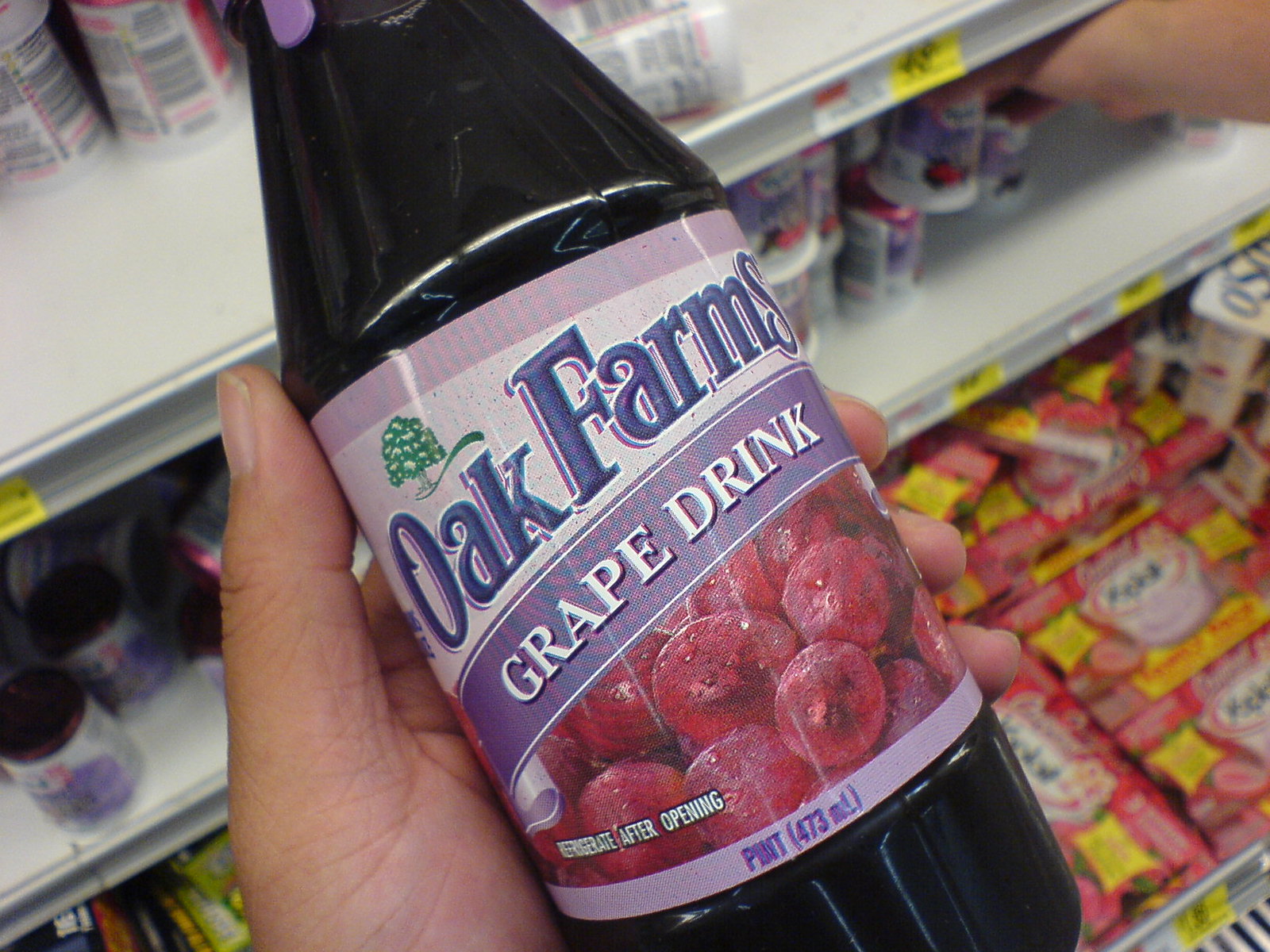A detailed caption for the image could be:

"In this vibrant image, a person is holding a bottle of Old Farms Grape Drink in a store, showcasing their thumb gripping the purple bottle while their fingertips wrap around the right side. The brand name 'Old Farms' is prominently displayed on the label, along with an inviting image of actual grapes beneath the clear text 'Grape Drink,' ensuring there's no confusion about the beverage inside. The bottle features a purple tab at the top for easy opening. The scene is set in a refrigerated aisle, evident from the silver shelving visible in the lower right-hand corner. Directly below the held bottle, multiple containers of yogurt are neatly arranged on the bottom shelf, including the recognizable Yoplait brand that another shopper is in the process of selecting from the display."